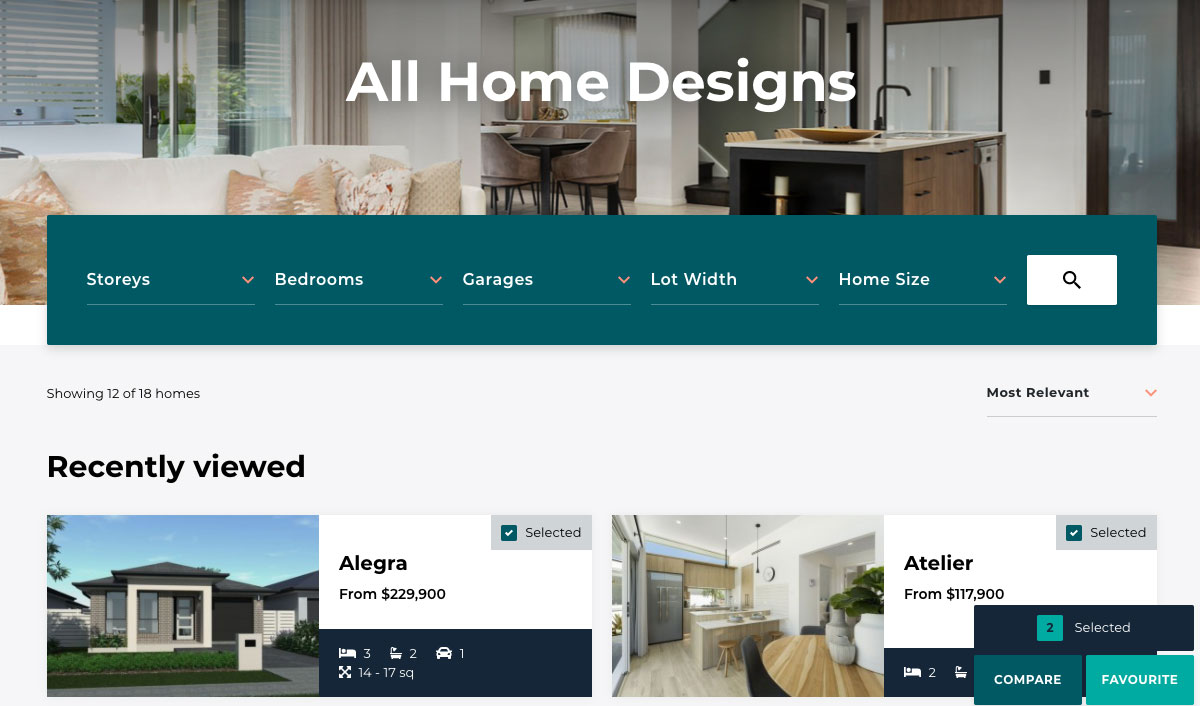A screenshot from a website titled "All Home Designs" showcases a modern living space bathed in natural light. In the background, large windows illuminate a beige couch positioned near a cozy kitchenette. The kitchenette features an island equipped for dishwashing. To the side, there is a door and a window offering additional sunlight and views of the outdoors. 

In the middle of the screenshot, a teal rectangular banner displays "Stories," "Bedrooms," "Garages," "Lot Width," and "Home Size" in white text. Adjacent to this banner is a white search box with a gray magnifying glass icon, indicating a search function. Below this, the site notes that it is "Showing 12 of 18 homes."

At the bottom of the screenshot, there are listings for various homes. A highlighted image shows a beige ranch house labeled "Allegra" with a price range from $229,900 to $229,900, marked as "Selected." Next to it, another home labeled "Adalia" is listed with a price starting at $117,900, also marked as "Selected." Both listings include teal buttons for "Compare" and "Favorite."